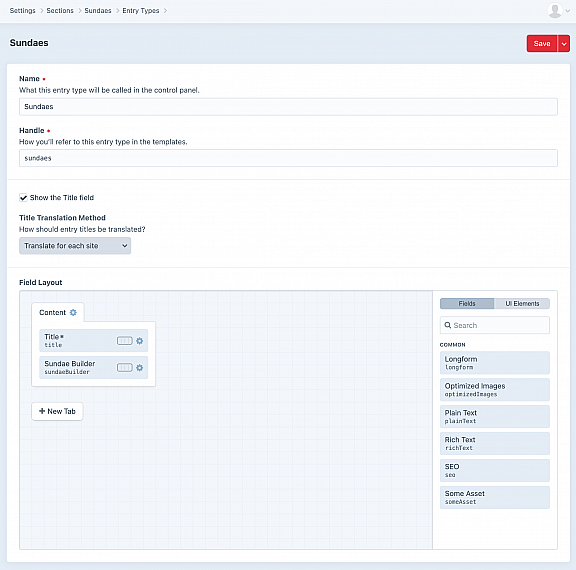**Detailed Caption for Website Settings Interface:**

This screenshot showcases the settings interface of a website, prominently featuring a section titled "Sundays." At the top-right corner, there's a drop-down menu for choosing a username. Directly beneath this, a red "Save" button with an adjacent drop-down menu is positioned.

To the left, under the "Settings" header, "Sundays" is emphasized in bold, appearing in larger and darker text than the rest of the headings above. Below this heading, a new, well-organized form appears within a large white box. The form begins with a "Name" field marked by an asterisk to indicate it is mandatory. 

Following the name field is an entry type field, labeled "What is this entry type called in the control panel?" It currently displays "Sundays," but offers the flexibility to change it. Below, the "Handle" field, also marked with a red asterisk, indicates how this entry type is referenced in templates; in this case, it is "sundays" in all lowercase.

A faint line divides these initial form fields from subsequent sections. The next portion contains a checkbox labeled "Show the title field," followed by the "Title Translation Method" heading in bold, asking "How should entries be translated?" with a corresponding drop-down menu offering options such as "Translate for each site."

Another separating line leads to a section titled "Field Layout," highlighted in a blue box with "Content" beneath it. This area includes a "Title" field with an asterisk, a checkbox (currently unchecked), and a lowercase "title." Additionally, there is a "Sunday Builder" option in lowercase, accompanied by another new tab feature titled "Field."

On the far right side of this interface, a tab labeled "Field" is currently active, alongside a search function. Below this, various common sections are listed: "Long Form," "Optimized Images," "Plain Text," "Rich Text," "SEO," and "Some Asset." Beyond the fields, there are several unselected UI elements.